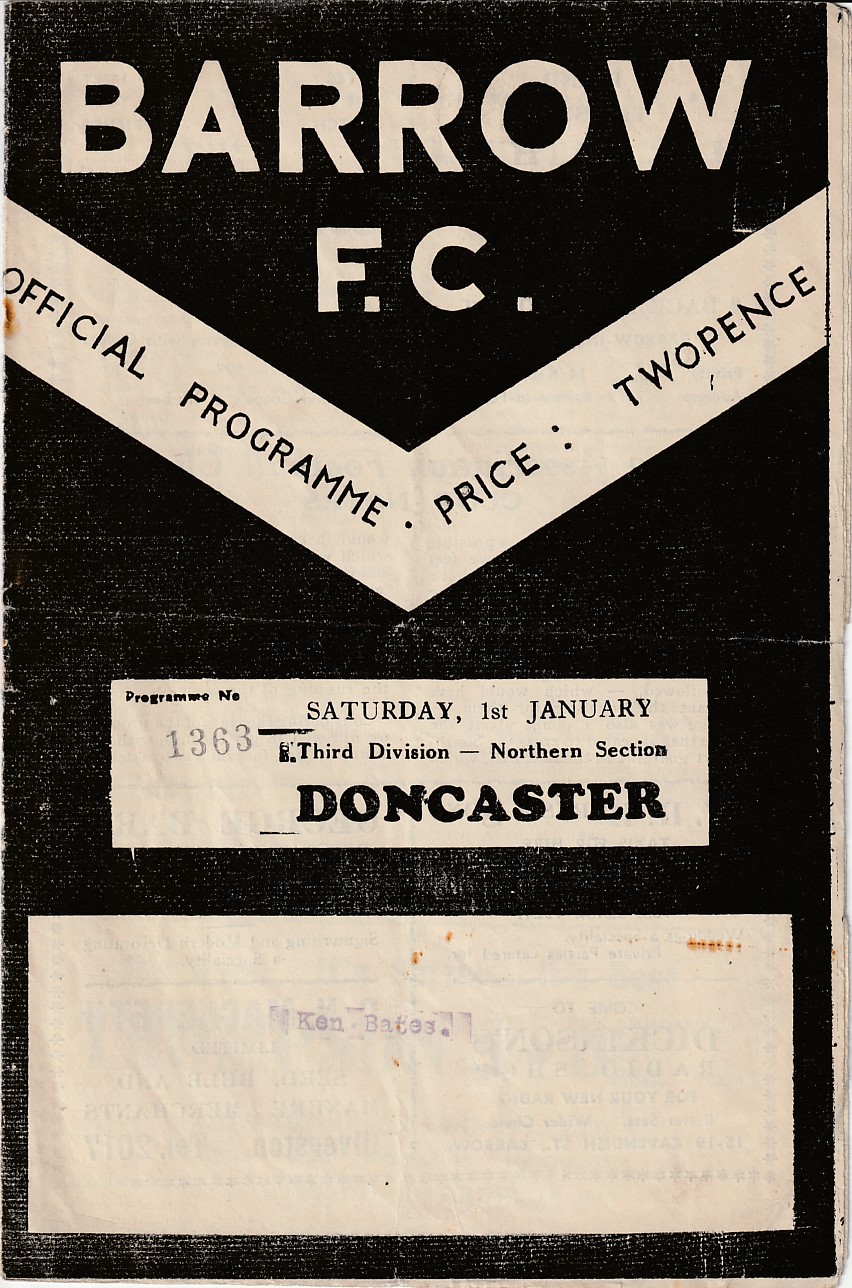The image depicts an official program, likely for a sporting event, designed with a brown background and beige text. At the top of the long rectangular page, the word "BARROW" is prominently displayed in large capital letters. Below it are the initials "F.C." separated by small square dots. The program features a V-shaped banner that reads "OFFICIAL PROGRAMME" in smaller, thinner capital letters, followed by "PRICE: TWO PENCE."

Further down, the content details Saturday, 1st January, describing it as the "3RD DIVISION NORTHERN SECTION," with "DONCASTER" boldly highlighted below. In the lower-left corner, the program number "1363" is stamped. At the bottom, there is a large rectangular section in beige, with some faded, unreadable text and a small red-stamped mark in the upper right corner.